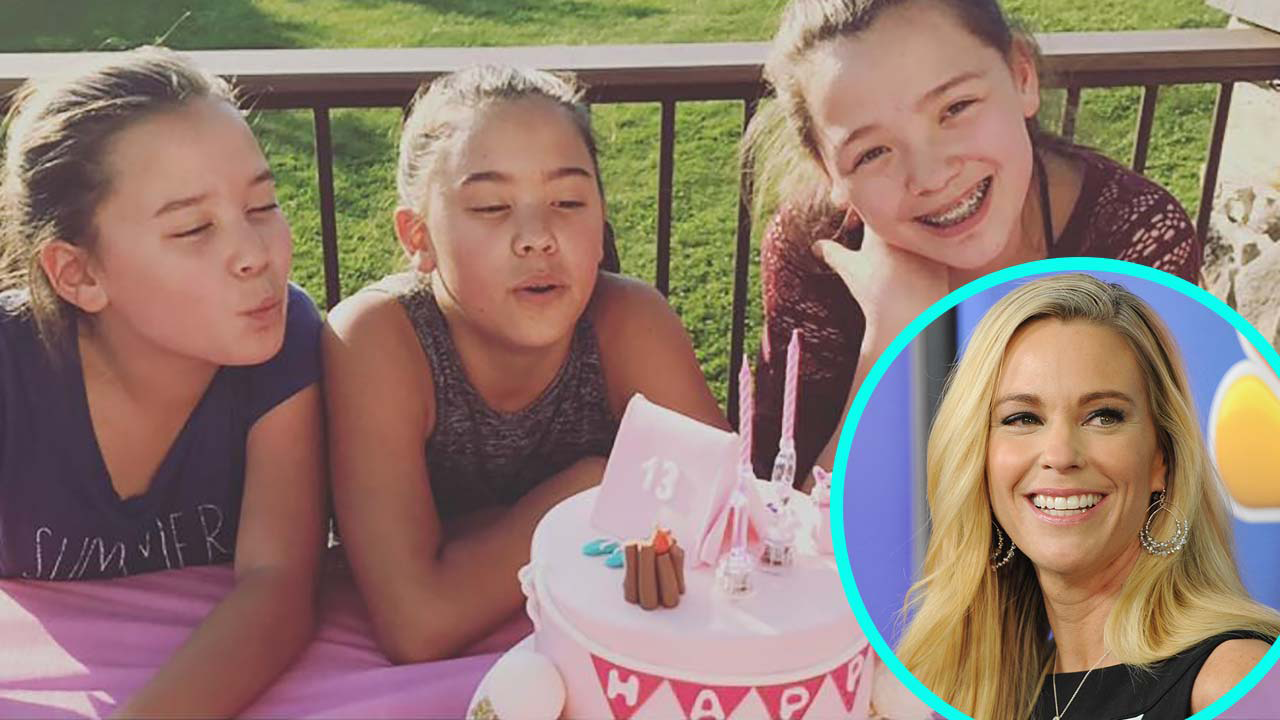In this vibrant and heartwarming photograph, we see three young girls, likely aged 12 to 13, celebrating a 13th birthday on an outdoor deck with a manicured green lawn in the background. The girls appear to have mixed Asian and Caucasian heritage, and are gathered around a pink birthday cake adorned with the words "Happy Birthday" and the number 13, along with a few pink candles. Two of the girls, who seem to be twins, are captured in the moment of blowing out the candles, while the third girl, with braces, is beaming a beautiful smile at the camera. They are dressed in summer attire, with one wearing a tank top and the other in a short-sleeved shirt. The festive scene is completed by a pink tablecloth. Additionally, there is an inset circular image of an attractive blonde woman with a radiant smile, who appears as if she could be a host or a character from a TV show, adding a promotional twist to the birthday photo. This seamless blend of celebration, youth, and warmth makes the image a joyful capture of a significant milestone.